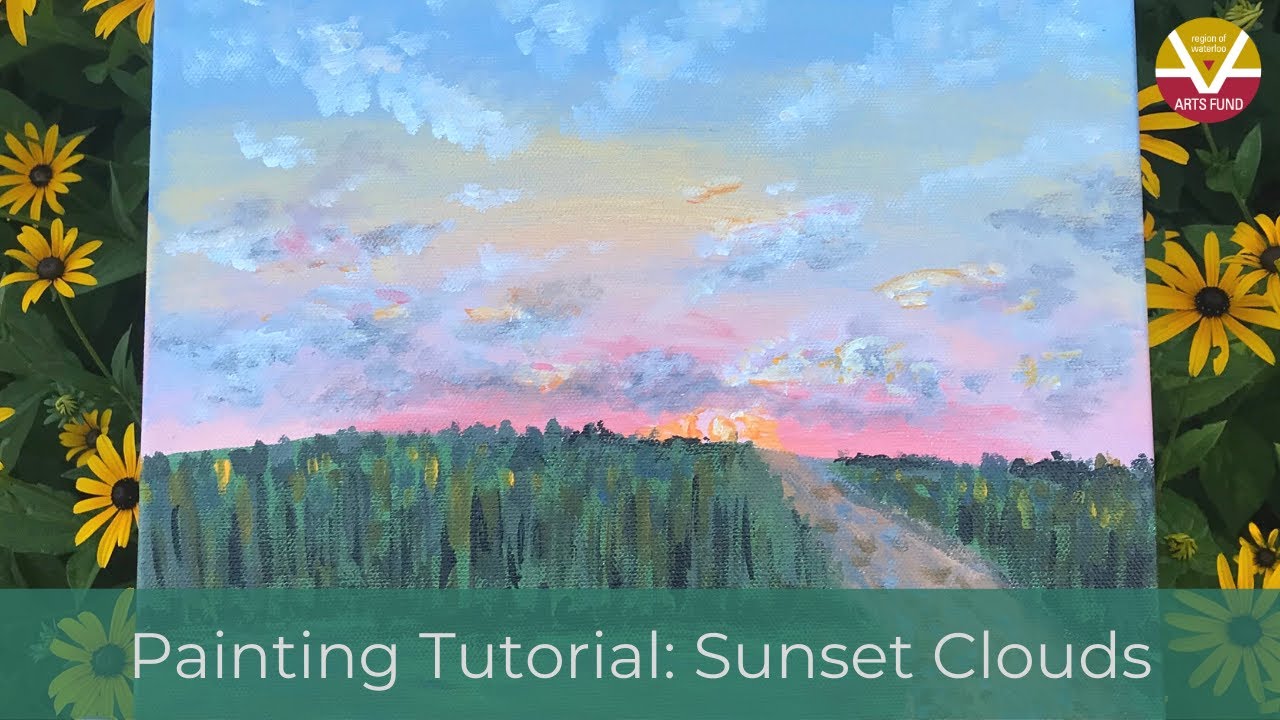The image is an advertisement for a painting tutorial titled "Sunset Clouds" featuring a detailed watercolor or acrylic painting. The painting depicts a serene sunset scene with a forest and a winding dirt road leading towards the horizon. The sky showcases a stunning gradient of bubblegum pink, blue, and hints of yellow and purple with scattered clouds. The foreground of the image includes fields of greenish-blue grass flanking the road. In the background, the painting is juxtaposed against either an image or another painting of bright yellow flowers with dark centers, likely daisies, adding depth and contrast.

The painting tutorial text is displayed at the bottom of the image in white letters against a translucent green background. This text clearly reads "painting tutorial: sunset clouds." The top right corner of the image features a circular logo that says "Region of Waterloo Arts Fund," highlighting the source of the arts funding and support. The overall composition, with its vibrant colors and intricate details, creates an inviting and educational visual experience for viewers interested in the art of painting landscapes.